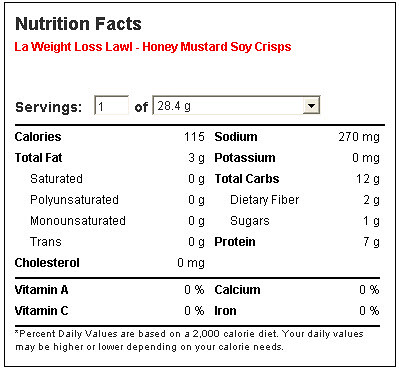The image displays a food label against a white background, framed by a black outline. At the top, "Nutrition Facts" is prominently printed in bold black lettering. Directly underneath, smaller red letters spell out "L.A. Weight Loss L.A.W.L-Honey Mustard Soy Crisps."

The label is divided into detailed sections, beginning with serving size information: "Serving Size: 1 of 28.4 grams."

Nutritional information is meticulously itemized below:

- **Calories:** 115
- **Total Fat:** 3 grams
  - **Saturated Fat:** 0 grams
  - **Polyunsaturated Fat:** 0 grams
  - **Monounsaturated Fat:** 0 grams
  - **Trans Fat:** 0 grams
- **Cholesterol:** 0 milligrams
- **Vitamin A:** 0%
- **Vitamin C:** 0%
- **Sodium:** 270 milligrams
- **Potassium:** 0 milligrams
- **Total Carbohydrates:** 12 grams
  - **Dietary Fiber:** 2 grams
  - **Sugars:** 1 gram
- **Protein:** 7 grams
- **Calcium:** 0%
- **Iron:** 0%

At the bottom, a standard disclaimer states: "*Percent Daily Values are based on a 2,000 calorie diet. Your daily values may be higher or lower depending on your calorie needs.*" This ensures consumers are aware of the relative quantities based on their individual dietary requirements.